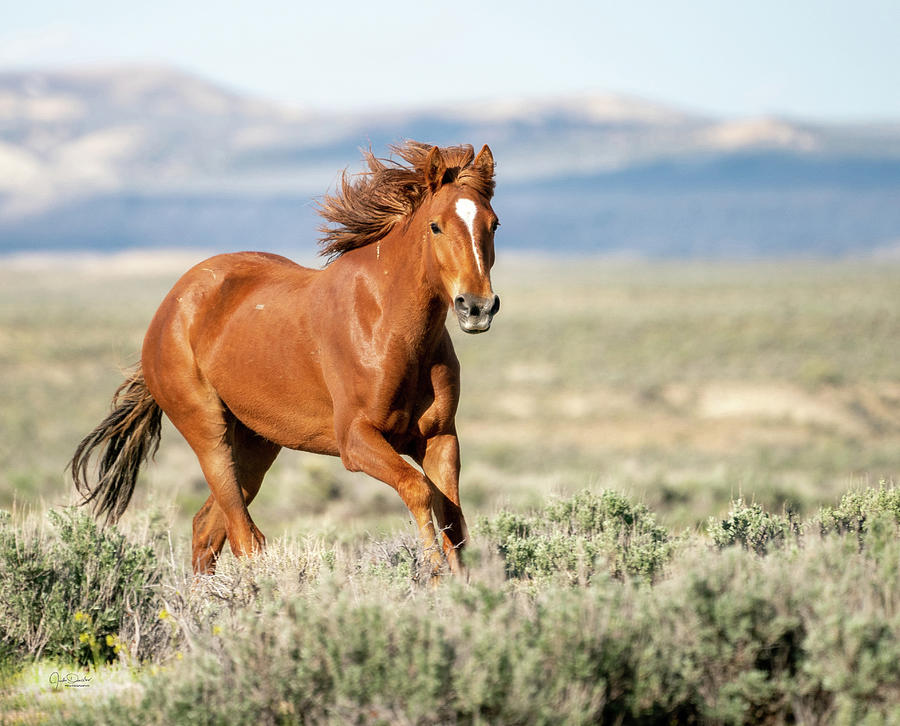This professionally shot, high-quality image captures a glossy, chestnut horse mid-trot, galloping through an expansive, open grassland. The young horse, possibly between two to five years old, exhibits a strikingly shiny, orangish-brown coat with a similarly colored mane and tail. A distinctive white stripe runs down its face from the center of its eyes to near its nose, accentuating its classic equine appearance. 

The horse, a muscular and powerful figure reminiscent of a wild mustang, faces the photographer directly, suggesting it is turning slightly to its left as it moves. The photo is well-lit, indicating it was taken during mid-afternoon. The foreground is slightly blurred, directing the viewer's focus to the horse, while the background features the further blurred outline of prairie-like plains or potentially low mountains, adding depth and context to its natural and rural setting. The ground is a mix of green and gray grasses interspersed with some dead weeds and shrubs, painting a vivid picture of the meadow or prairie landscape that the horse traverses. The image skillfully conveys the dynamic motion and vitality of the horse within its serene environment.